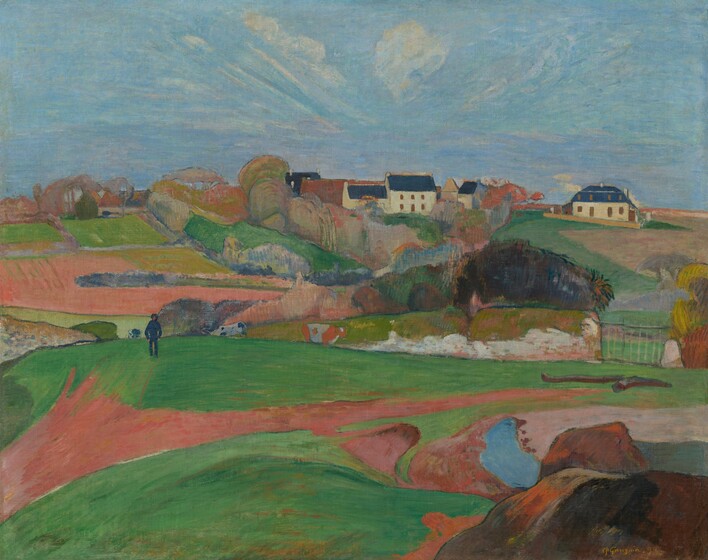This image appears to be a painting or a drawing, possibly executed with colored pencils or chalk. Its style is reminiscent of Van Gogh but unidentified due to an indistinct signature in the lower right corner. The rectangular artwork measures approximately six inches wide by four inches high. The scene captures a picturesque hillside, covering the bottom two-thirds of the image with the sky occupying the top third.

The sky is depicted in shades of light blue with a mix of thinner clouds and one prominent large, fluffy white cloud. Below, the landscape is diverse, featuring a series of tilled and cultivated fields in hues of brown, green, and yellow-gold, separated by rows of hedges and bushes. At the summit of the hill, several white houses with slanted blue roofs stand against the horizon, possibly part of a single compound or multiple properties.

A figure dressed in a dark blue outfit walks along a green lawn in the lower left part of the painting, with a few cows grazing nearby. Their presence, though not the focal point, adds a human element to the serene rural setting. Gates and paths interweave through the farmland, hinting at access to the buildings.

In the foreground, the scene captures additional details, including tall rocks, what seems to be a small blue pond, and stretches of green grass and dirt roads. The overall composition, with its melding of vivid agricultural life and tranquil skies, creates a vivid yet subtly detailed portrayal of rural charm.